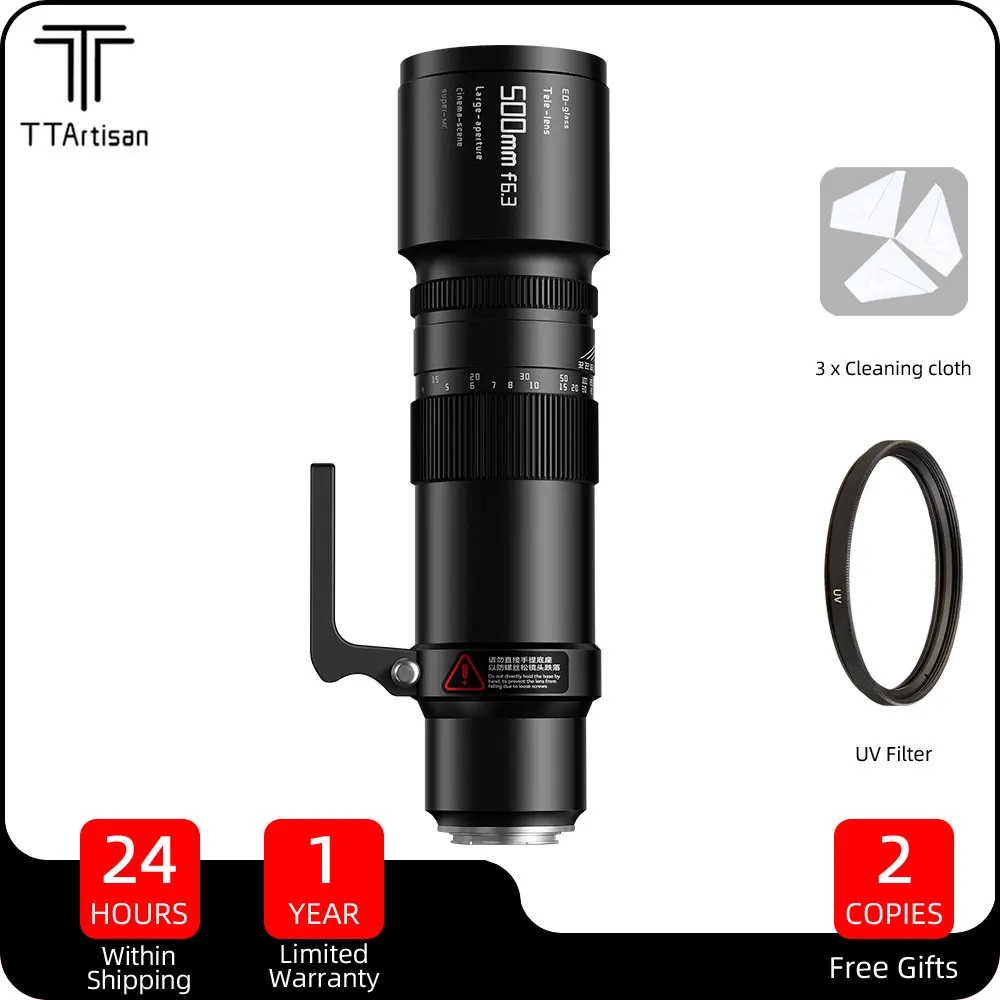This is a highly detailed infographic image of a TT Artisan camera lens set against a white background. The lens, which is labeled as 500mm f/6.3, appears in a shiny black cylinder reminiscent of a compact telescope or a piece of binocular equipment. At the top left, the brand logo "TT Artisan" is displayed prominently. To the right of the lens, the image lists "3x Cleaning Cloth" alongside a small image of cleaning cloths on a gray background. Below this, it shows "UV Filter" illustrated with the black edges of a filter lens. At the bottom of the image, several pieces of numerical information are presented within a red background: "24 hours" likely indicating expedited shipping, "one year" referring to a limited warranty, and "two copies," possibly indicating a special offer or package contents. The overall design suggests it is a product listing commonly found on online shopping platforms.